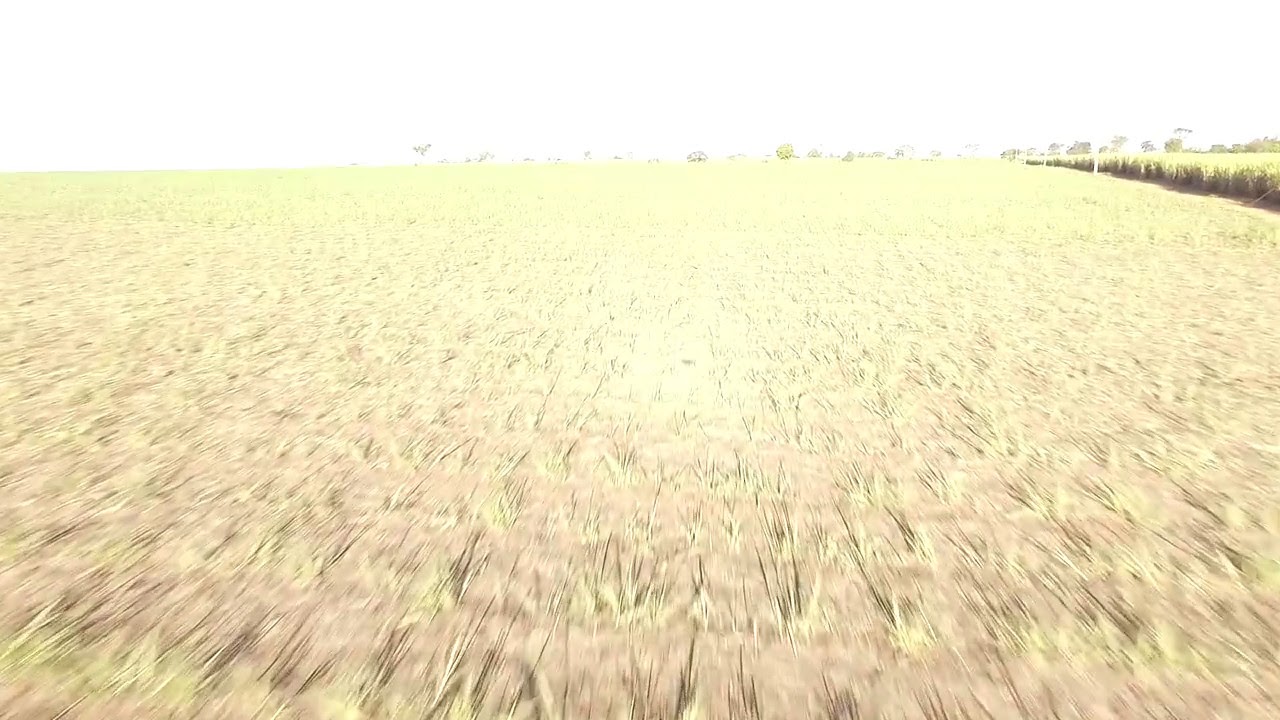This image, likely a screenshot from a video taken from an aircraft, depicts a large agricultural field from a top-down perspective. The scene appears to be in motion, as if the viewer is flying swiftly over the field, causing a blur that obscures fine details. The field itself is a mix of yellow and brown hues, suggesting ripened crops such as wheat. The earth is carved into furrows with spiky green and white plants standing amid the blurred motion. On the right side of the image, the field gives way to a road separating it from another field where taller, thickly grown plants, possibly similar crops, stand. The distance reveals diminutive-looking trees, shrunken only by perspective. The entire image is washed out by intense light, rendering the sky and parts of the background as a featureless white expanse.